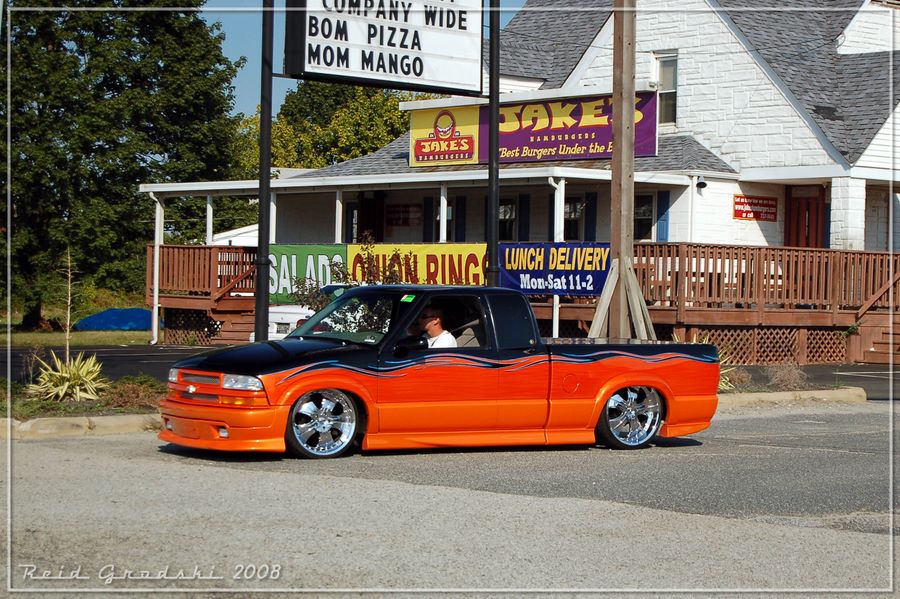This vibrant landscape photograph captures a heavily modified lowrider pickup truck, likely a Chevy S10, in the foreground as it cruises down a cement street. The truck features a striking two-tone paint job, with the bottom half in a bright fluorescent orange adorned with a flame design where it meets the dark navy blue, possibly black, upper half. The vehicle is equipped with chrome five-star rims, approximately 18 inches in size, and sits extremely low to the ground, nearly scraping the pavement. A man in a white t-shirt and sunglasses confidently navigates the truck.

In the background, a bustling small-town restaurant named "Jake's Best Burgers" is visible, characterized by its white walls and a roof with gray shingles. The restaurant sports a large, colorful sign in purple, red, and yellow, although partially obscured, promoting its offerings. Surrounding the establishment is wooden fencing adorned with various promotional signs including one advertising "Salads" in white text on a green background, another showcasing "Onion Rings" in red text on a yellow background, and a third promoting "Lunch Delivery" with blue and yellow text. Additional elements in the background include the calm surface of a man-made lake and a few scattered trees, particularly on the left side of the image.